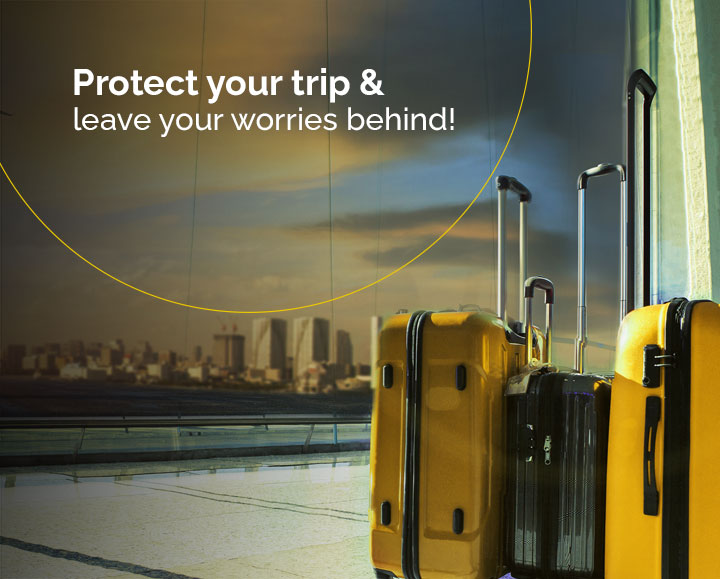In vibrant white bold font, the phrase "Protect Your Trip" stands out over a scenic backdrop, immediately catching the viewer's attention. Just beneath, an inviting message, "Leave Your Worries Behind," arcs elegantly in a gold or yellow hue. The image captures a scene from a high vantage point, perhaps a rooftop or airport tarmac. Three black suitcases, towering and sturdy with their pull handles extended, are meticulously lined up, symbolizing travel readiness and security. In the background, an urban skyline of imposing skyscrapers suggests the bustling city of departure. Dark, ominous clouds loom overhead, creating a stark contrast and invoking a sense of looming concern. The overall composition conveys the necessity and reassurance of trip insurance, ensuring peace of mind and the promise of a worry-free, enjoyable journey despite potential challenges.